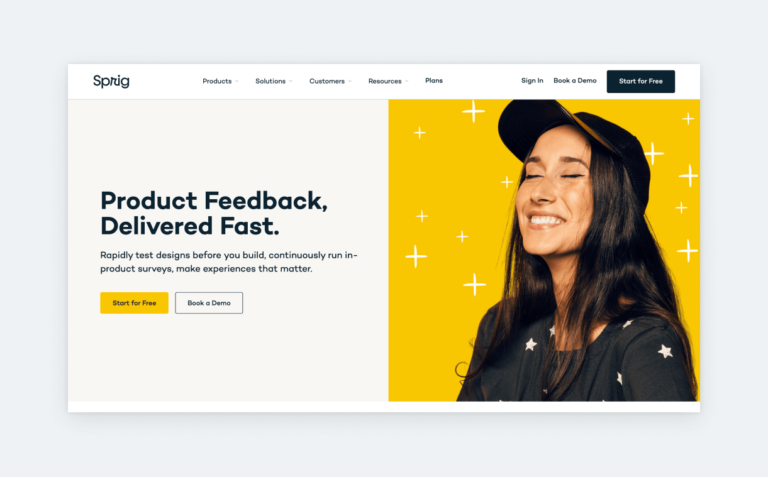This is a screenshot from a software interface named Sprigg. The top-left corner features the logo "Sprigg" in dark grey uppercase letters. Adjacent to the logo, there is a navigation menu listing options: Products, Solutions, Customers, Resources, and Plans. Further to the right, there are buttons for "Sign In" and "Book a Demo," as well as a prominent "Start for Free" button in white text on a very dark grey, almost black tab.

The screen is divided into two sections. On the right side, there is a dark yellow square adorned with white plus symbols in the background. In the foreground, a woman is seen smiling with her eyes closed, captured in a side profile with her left side facing the camera. She has a radiant smile, wears a black ball cap, and has slightly tanned skin. Her long, straight dark brown hair cascades over her shoulders, and she dons a black top with white star patterns.

The left side of the screen features the text: "Product feedback delivered fast. Rapid test designs before you build, continuously run in-product surveys, make experiences that matter." Below this, there are options to "Start for Free" or "Book a Demo."